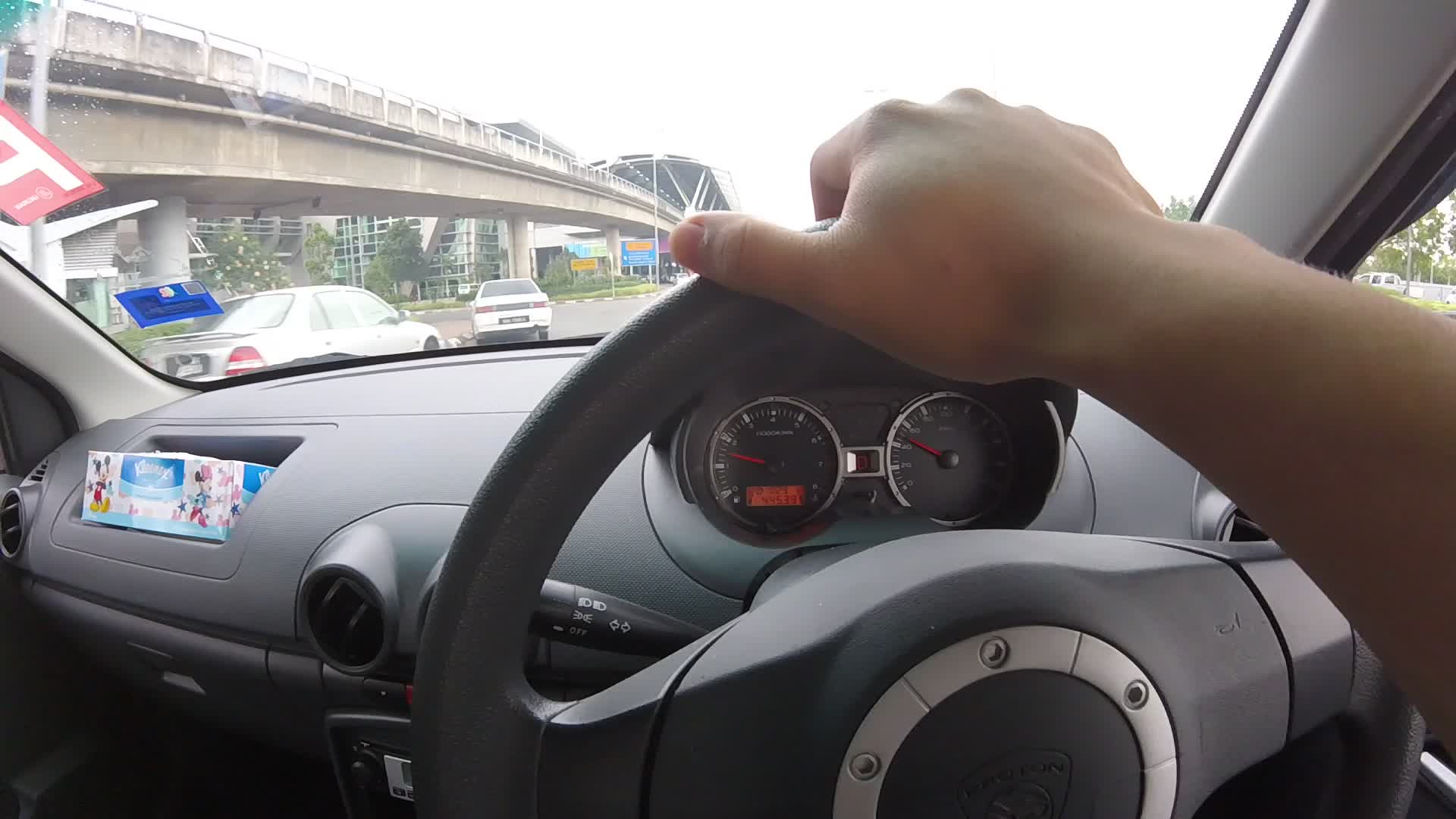The photo captures an interior view of a compact car from the driver's perspective, emphasizing the driver's right hand gripping the gray plastic steering wheel, positioned at the top. On the gray dashboard, just above the glove compartment, rests a Disney-themed box of Kleenex featuring Mickey and Minnie Mouse. The car appears to be driving in England, indicated by the right-hand driving position and the visible license plates of the two white cars ahead, one of which is making a left turn. Outside, a bridge runs along the left side of the road, possibly leading to a station or an overpass, hinting at a freeway on-ramp or an airport parking area. The sky is notably bright yet overcast, casting a grayish-white hue over the scene. The driver's arm, with a dark brown skin tone, suggests that the individual may be of Middle Eastern or Indian descent.